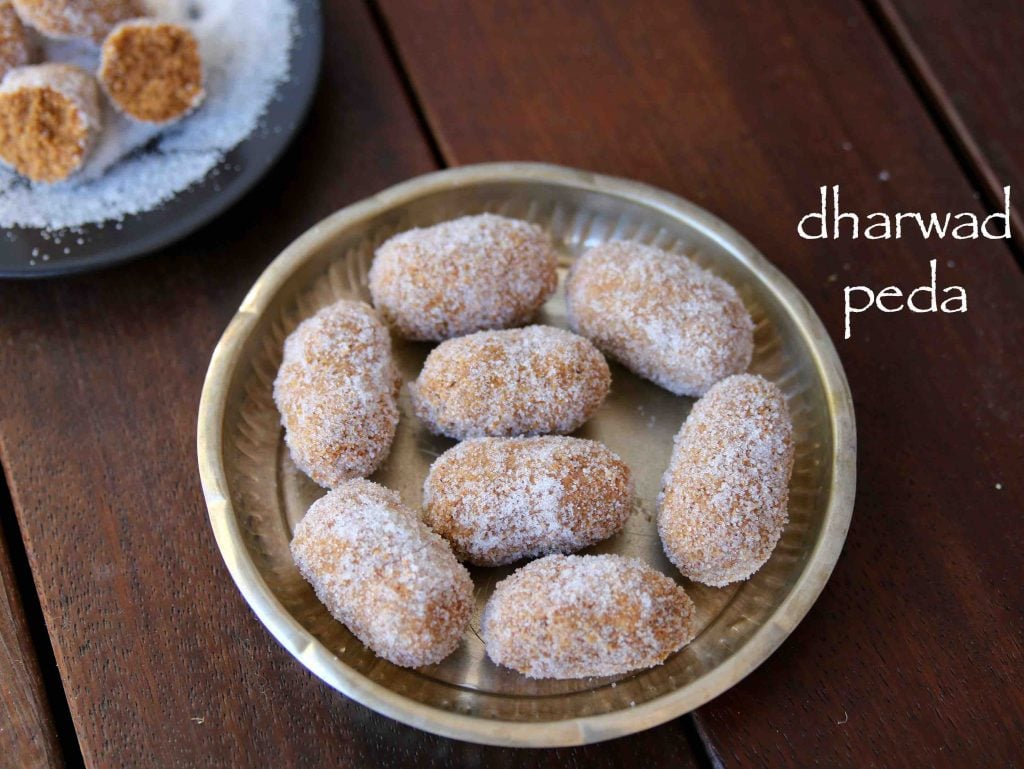Displayed on a dark mahogany wood table, this wide vertical rectangular image showcases a circular silver dish with vertical indentations around its sides. Inside the dish, there are eight puffed, oval-shaped treats, light brown in color and generously dusted with powdered sugar. These treats are arranged in a circular pattern with two positioned side-by-side in the center. To the left edge of the image, in the top corner, one of these treats is shown broken open, revealing a darker brown interior. In the top right of the image, the text "dharwad pedha" is written in white.